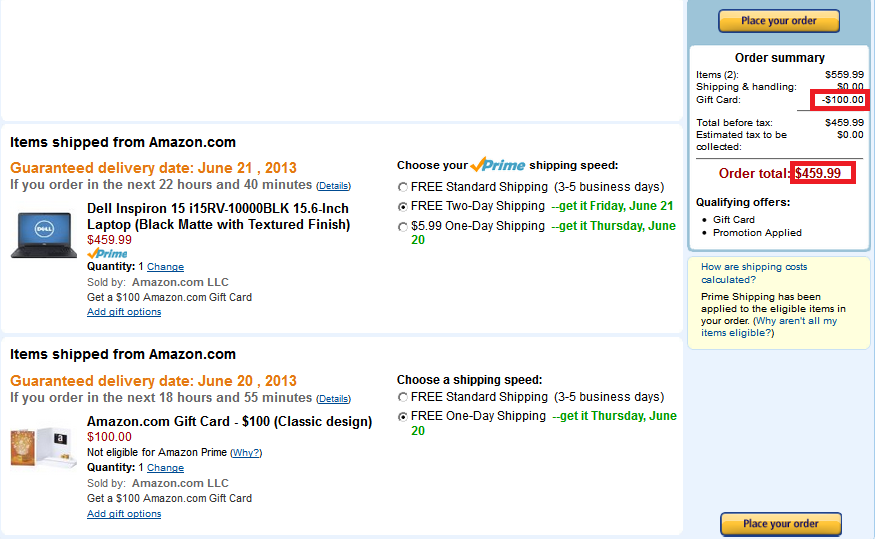The image depicts the checkout page on the Amazon.com website, detailing the purchase of two items. The first item is a Dell Inspiron 15 laptop priced at $459.99, eligible for Prime shipping with an expected delivery date of Friday, June 21st. The second item is a $100 Amazon gift card, available for free one-day shipping with an expected delivery date of Tuesday, June 20th.

On the right side of the page, there is a panel featuring two prominent yellow buttons labeled "Place your order." Above these buttons is an order summary indicating the purchase of two items totaling $559.00, with no charges for shipping and handling. There is a $100 deduction for the gift card, highlighted in a red box. The total before tax is listed as $459.00, with an estimated tax of $0.00. Consequently, the order total amounts to $459.99. Below this total, a note specifies that qualifying orders and promotions have been applied, with this section also highlighted in red. The background color of the website is white.